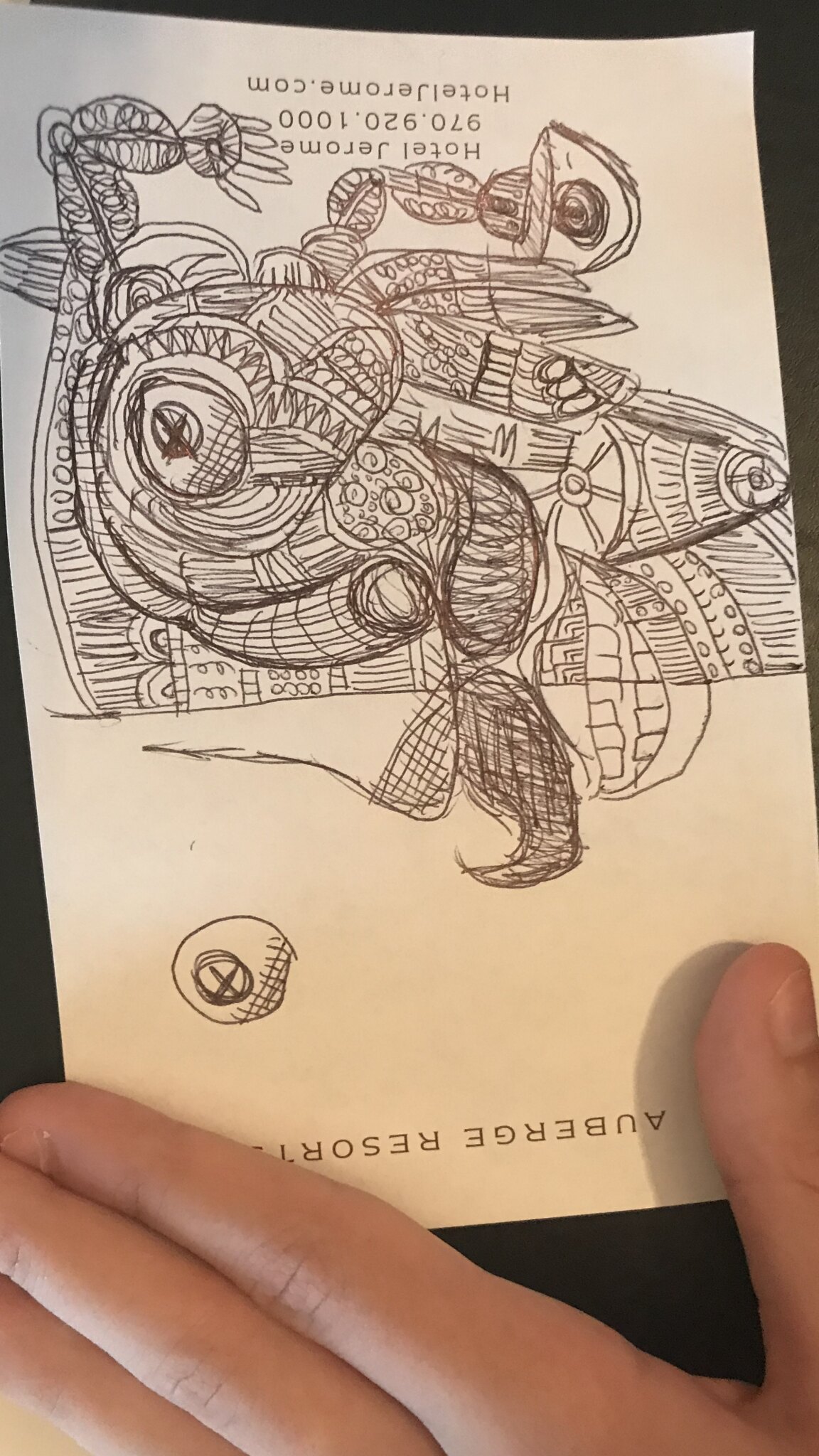This photograph features an intricate line drawing held by a person with light-colored skin. The person's thumb and three fingers are visible at the bottom edge of the paper, suggesting they are holding it. The drawing itself is oriented upside down in the image, adding to its complexity. The artwork appears to be rendered in brownish or black pencil, with lighting that imparts a yellowish tone to the paper. 

Upside down text at the top of the drawing seems to read "Aubergé" and "Pessori," though it is challenging to decipher. The detailed illustration prominently features various eyes intermingled with an array of mechanical components and tendrils, creating a surreal and complex design. Some elements stand out, such as an eye positioned atop a leg, another eye on a tendril to the right, and a random eye appearing at the bottom (which is the top in the image's orientation). The bottom of the drawing, which is at the top of the photo, contains additional writing that remains unreadable due to its inverted position. The background is entirely black, providing stark contrast to the detailed, lighter drawing.